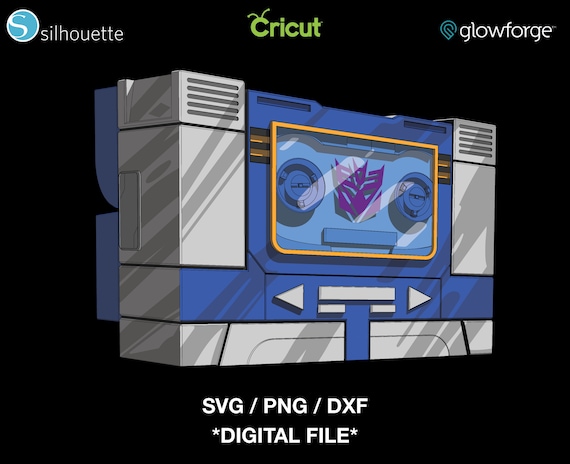The image showcases a detailed, computer-aided illustration of a rectangular cassette player, approximately three inches high and four inches wide. The player features a Transformers Decepticon symbol — a contrast to the noted Autobot in the description — prominently in its center within the tape area. The cassette player is primarily blue and gray, accented with a gold trim around the tape area. Additional decorative elements include left and right arrows below the tape area. 

The entire scene is set against a plain black background. At the top of the image, three distinct logos are visible: on the upper left, “Silhouette” is written next to a light blue circle with a white 'S'; in the top center, “Cricut” is displayed in bold green text, complete with antennae extending from the first 'C'; and on the upper right, “Glowforge” is presented in white text beside a blue 'G' logo. 

Beneath the cassette player, two lines of text in white read, “SVG/PNG/DXF” on the first line and “*digital file*” on the second line. This intricate assembly of design elements and transformative symbology is presented within a precise illustrative frame.